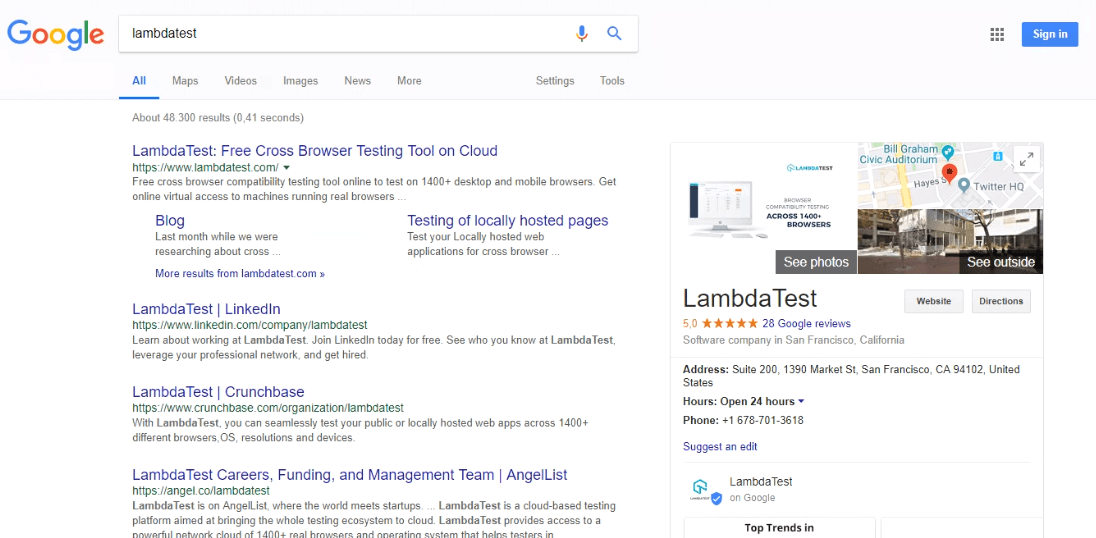A user conducted a voice search for "LambdaTest" as one word, combining the Greek letter "Lambda" and "test." The search returned four primary links: 

1. LambdaTest.com - Described as a free cross-browser testing tool on the cloud.
2. LambdaTest's LinkedIn profile.
3. LambdaTest on CrunchBase.
4. LambdaTest on AngelList (angel.co).

On the right side of the search results, the physical location of their headquarters is listed in San Francisco, with an area code beginning with 678. Additionally, LambdaTest boasts a five-star rating from 28 Google reviews. The initial link elaborates on their service, mentioning free cross-browser compatibility testing for both desktop and mobile platforms, implying its use for testing how websites perform on various browsers like Firefox and others.